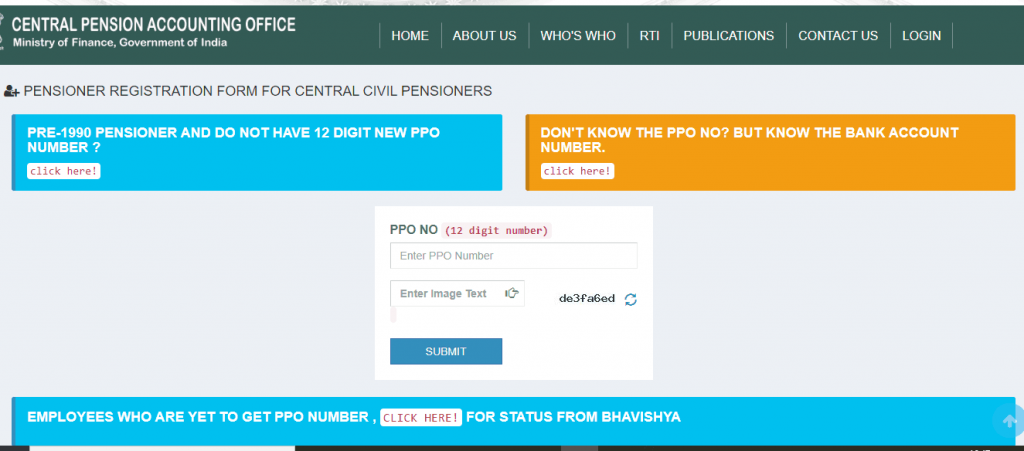The image features a structured webpage layout designed for the Central Pension Accounting Office. At the top of the page, there is a green rectangle containing the title "Central Pension Accounting Office." Below this header, the navigation menu appears in a sequence of white lines separating different sections. The menu options, easily identifiable, include "Home," "About Us," "Who's Who," an indiscernible item (possibly abbreviated as RH), "Publications," "Contact Us," and "Log In."

Midway down the page, there is a prominent blue rectangle featuring an icon of a person with a plus sign, indicating a link to the "Pensioner Registration Form for Central Civil Pensioners." Within this blue rectangle, a white button labeled "Click Here" invites action. Alongside this, an orange rectangle also contains a call-to-action button with the text "Click Here."

Further down, a white input field marked "PPO NO" is accompanied by some red text instructions. Two gray-outlined rectangles provide additional input fields, each containing some small text and an unclear symbol at the end of the second field. A blue "Submit" button is positioned immediately below these input sections.

On the right-hand side, there is a circle with arrows, potentially indicating a refresh or repeat action. At the bottom of the page, another blue rectangle addresses employees who have yet to receive their PPO number. This section instructs users to "Click Here" in red text within a white button to check their status on the BHAVISHYA platform.